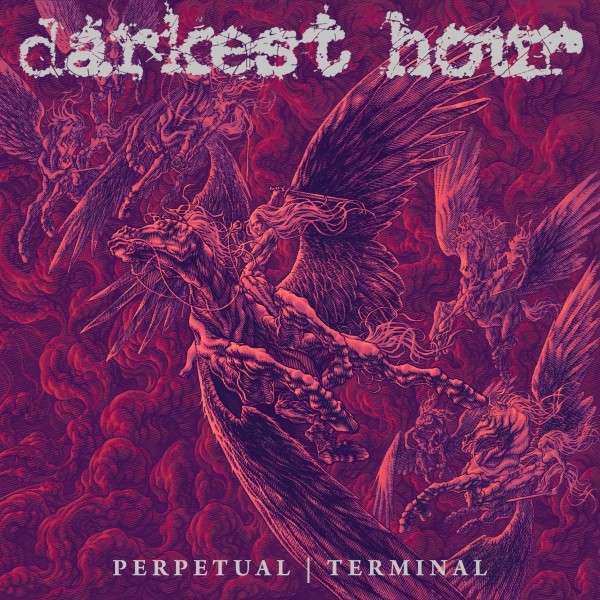The album cover for "Darkest Hour" titled "Perpetual Terminal" features a highly detailed, monochromatic image dominated by deep shades of red and burgundy, with intricate line art in darker hues verging on purple. Central to the design is a woman wielding a sword, riding a winged horse, seemingly leading a charge into battle. Surrounding her are figures that might either be her comrades or pursuing opponents, all blending into the smoky, swirling background that adds to the intensity of the scene. The high level of detail in the smoky backdrop and mythical creatures, possibly dragons or griffins, makes it challenging to distinguish the specifics as they merge seamlessly with the red tones. The text, “Darkest Hour” and “Perpetual Terminal,” stands out in a light gray, bubble font, against the dark backdrop, clearly marking it as an album cover, likely for a rock or dark music genre.